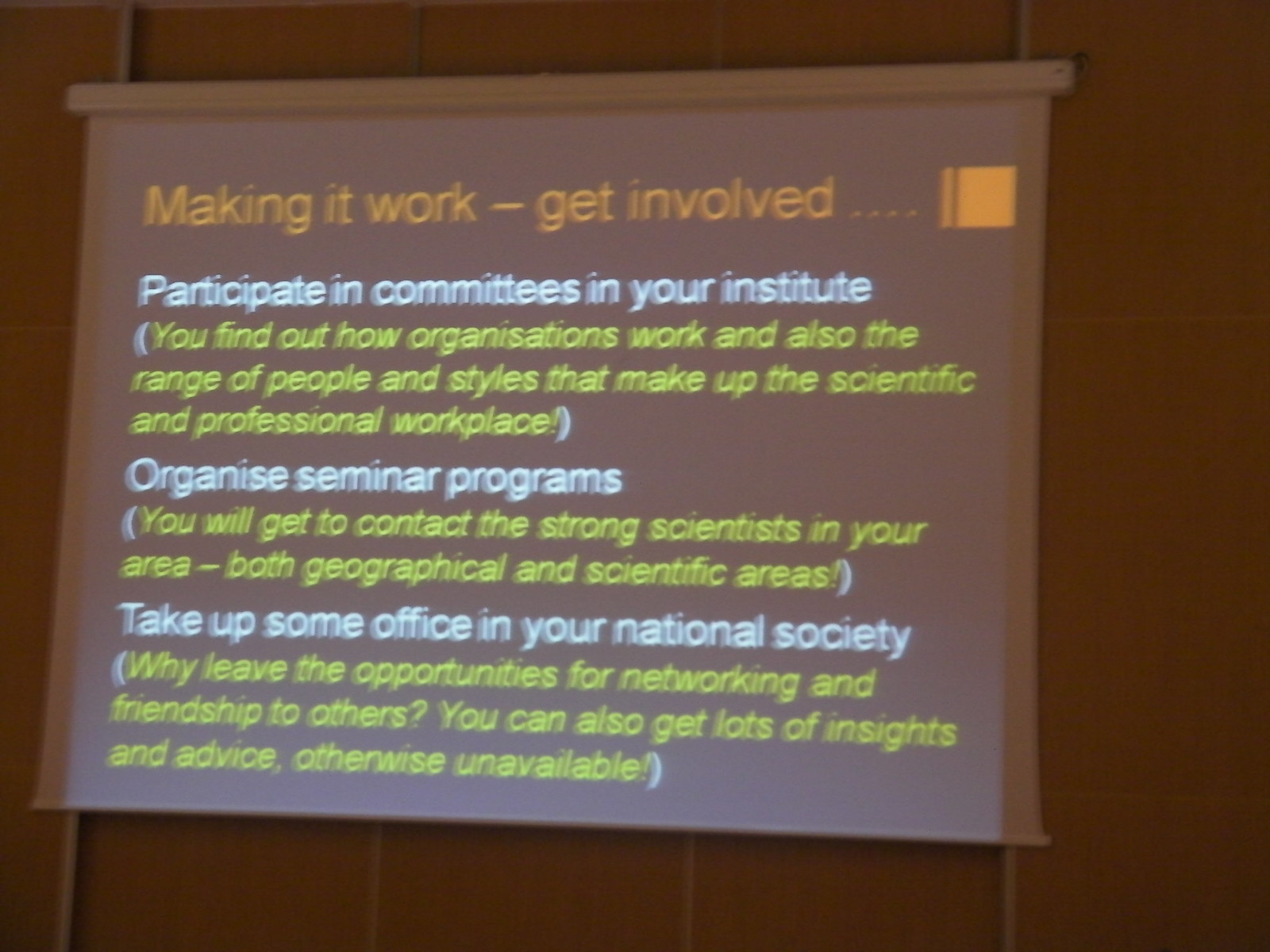The image features a projector slide with a brown background, displayed in a dim room. The slide, titled "Making it Work: Get Involved" in bold orange text, outlines various ways to engage in the scientific and professional community. The first point, in white text, encourages participation in committees within your institute, followed by a yellow annotation explaining that this helps understand organizational structures and the diversity of people and styles in the workplace. The next white text suggests organizing seminar programs, with a yellow note emphasizing the opportunity to connect with prominent scientists in both geographical and scientific areas. Then in white, it advises taking up an office in your national society, with a concluding yellow remark urging not to leave networking and friendship opportunities to others, highlighting the unique insights and advice that can be gained. The overall setting appears academic, given the dark room and focused content of the slide.